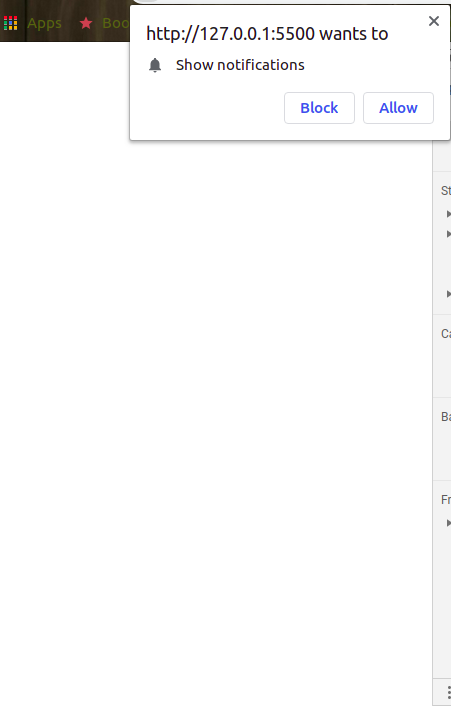The image displays a Google Apps interface featuring a rectangular popup notification. The popup is horizontally elongated with a white background. On the left side, it displays the URL "http://127.0.0.1". The popup includes two buttons labeled "Block" and "Allow," both designed with a white background, blue font, and a grey outline. In the upper right corner of the popup, there is a grey or black "X" button for closing the notification. The popup occupies roughly four-fifths of the image's width, leaving the rest of the screen in view.

In the upper left corner, there is a small, square section with a black background and a 3x3 grid of colored squares: three red squares at the top, followed by a green, blue, yellow, and another green square in the middle row, and two yellow squares with one empty space at the bottom. The word "Apps," written in dark green, is displayed alongside a red star and the word "BOO" in green. This section appears to be part of a thin navigation bar across the top. On the right side of the image, there is partial, illegible text starting with "FRMB."